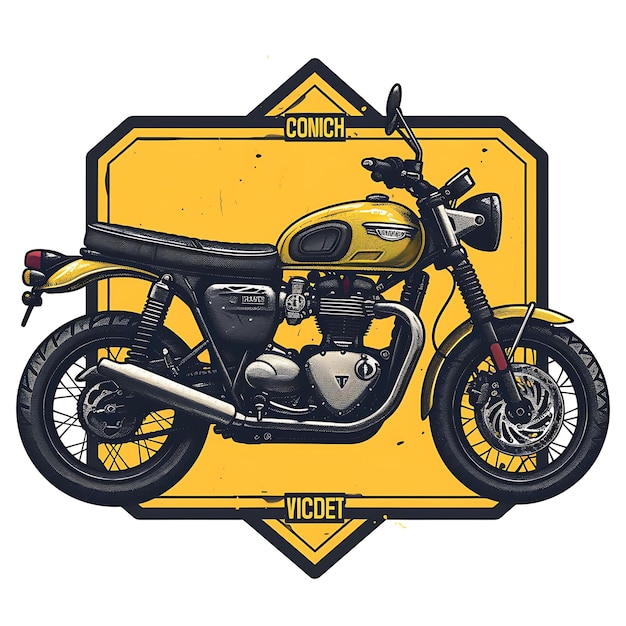The image is a digital artwork featuring an old-fashioned motorbike, reminiscent of the 1950s, predominantly in mustard yellow and black. The motorbike has distinctive yellow fenders and gas tank, with a metallic insignia on the tank area. It stands in front of a layered background of two yellow and black-bordered plates. The foremost plate is rectangular with the letters "CONICH" at the top and "VICDET" at the bottom. Behind this, a second plate appears at an angle, forming a diamond shape with visible triangles at the top and bottom. The motorbike has smaller wheels and a black seat, further accentuating its vintage charm.